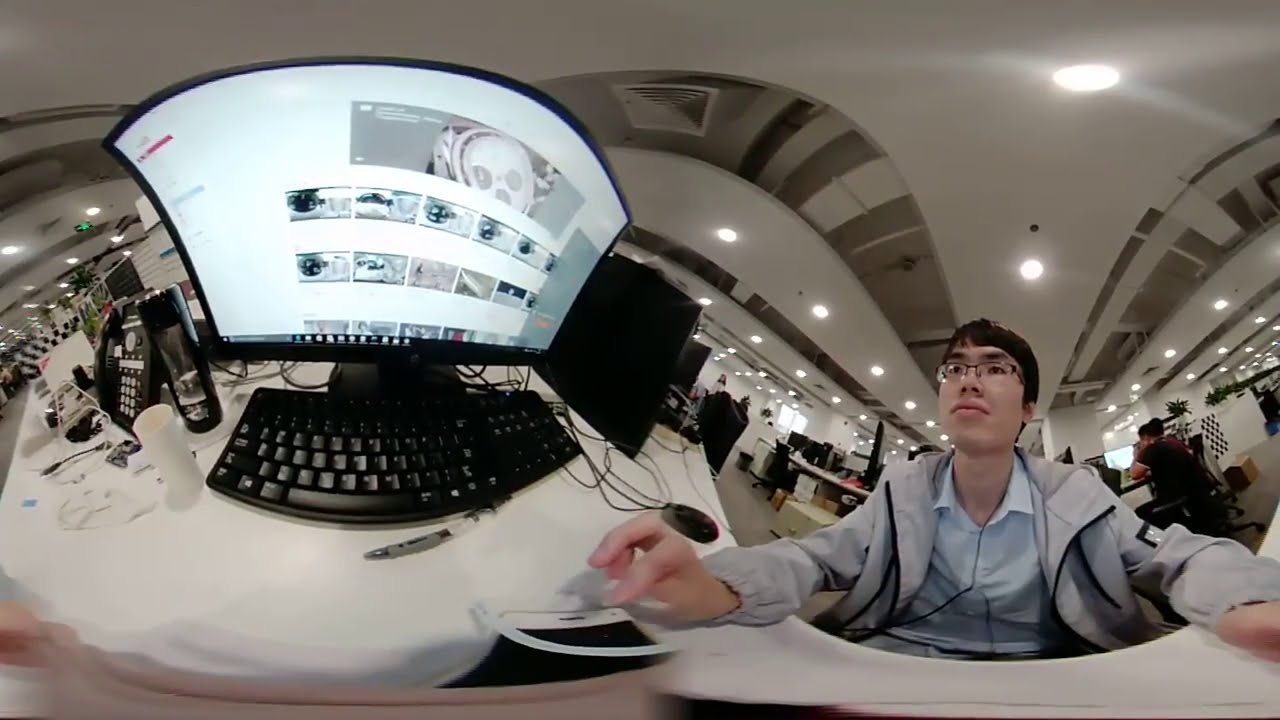The image, taken with a fisheye lens, captures a young Asian man with short black hair and glasses, seated at a desktop computer. He is wearing a blue shirt underneath a gray jacket, and appears to be either researching or watching videos online. The setting seems to be a large office building or possibly a university computer lab, as indicated by the presence of other people working at their own desks in the background. The man is also holding a smartphone, and his workspace includes various small items such as a pen, a cup, and a water bottle. Phones, computer desks, and numerous wires further suggest that the environment is bustling with activity typical of an office setting. The fisheye effect distorts the image towards the center, adding a unique, panoramic feel that captures the surrounding environment in its entirety.